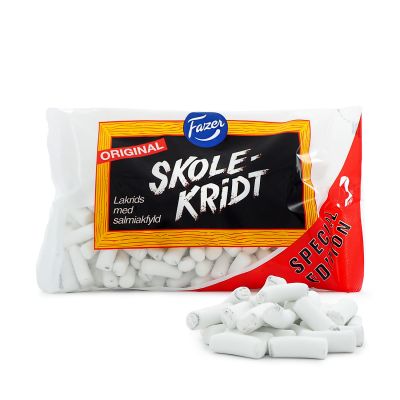The image depicts a clear plastic bag containing white, chalk-like candies that resemble small cylindrical pieces. The bag is predominantly white with a yellow border that frames the central area designed to look like a wooden frame. In the middle of this frame is a large black square. At the top of the bag, the brand name, "FAZER," is prominently displayed in white text over a blue circular logo with a distinctive curve below the brand name. The product, named "SKOLEKRIDT," is spelled out in individual letters within the black square. Below the product name, the word "ORIGINAL" is printed in white text on a red flag section. There's additional text, "Lækerhedsmed Salmæk Frid," in white at the bottom of the square, indicating that the language is likely of a European origin, possibly Norwegian. Situated at the bottom of the package in a red section, it states "Special Edition" in white text. In front of the bag, several of the white candies are displayed clearly, showcasing their resemblance to both chalk and cigarette butts, further suggesting their unique and possibly intriguing texture and flavor. The background of the image is plain white, focusing attention on the featured product.